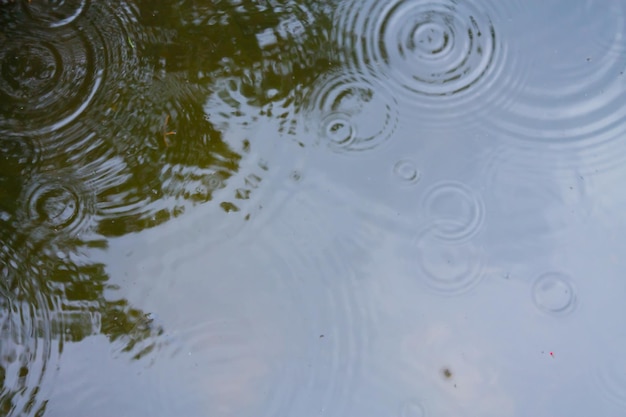A colored outdoor photograph captures a rain puddle on a street, viewed from above. The puddle, which has a shiny, oily sheen from engine grease, features roughly 12 to 13 raindrop impacts, each creating concentric ripples that spread outward. The water appears brownish due to the concrete beneath and is not clear enough to see below the surface. Reflections on the water's surface show the sky transitioning from bright blue in the lower right to darker blue in the upper right and a mix of green shades, suggesting tree limbs, in the upper left. The tree's reflection continues towards the lower left corner, indicating leaves that vary from bright to dark green. The image vividly captures the interplay of the rain with the urban environment and the natural reflections above.